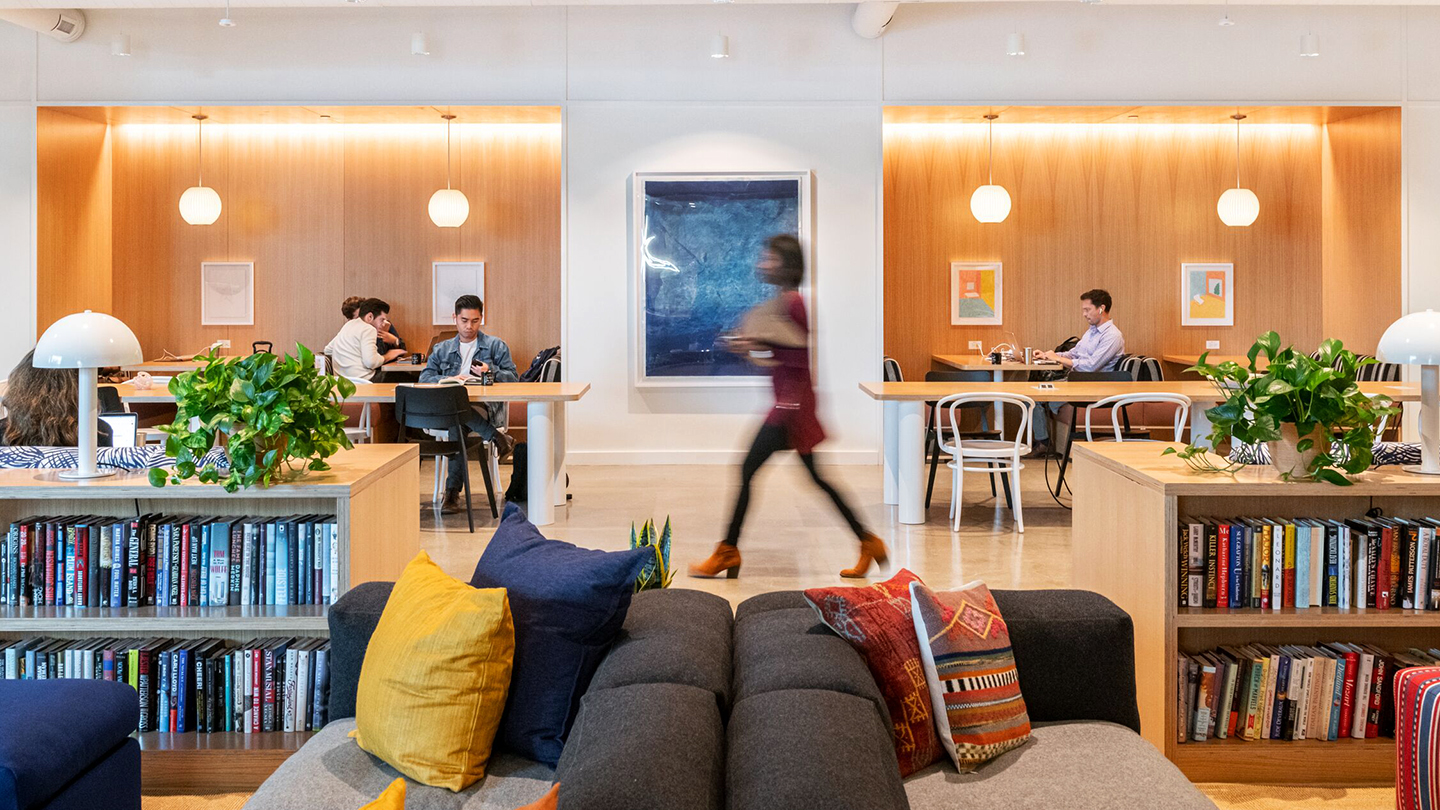The photograph showcases a modern, cozy space that could be a library or a cafe. In the center, there is a seating area featuring two sleek sofas with various colorful throw pillows ranging from gold, dark blue, orange, to red, and a mix of charcoal gray and light gray cushions. The left sofa has a navy blue and yellow pillow along with a beige blanket, while the right sofa features red and brown pillows. Flanking the sofas are two-shelf bookcases filled with vertically stacked books and potted artificial green plants atop them.

In the background, a light brown wooden wall is adorned with abstract artwork in hues of light and dark blue, and additional smaller framed pictures hang symmetrically on either side. Circular pendant lights hang overhead, contributing to the inviting atmosphere. Tables are scattered in the background where individuals are either reading books or working on laptops. There are about three people to the left and one to the right, engaging in various activities. The tables are light brown with chairs featuring steel frames in white and black.

A blurred woman in orange high heels and a dark crimson blouse is seen walking in the middle of the photograph, adding a dynamic element to the otherwise still image. Overall, the composition and elements suggest a well-designed, multi-functional space that encourages both relaxation and productivity.